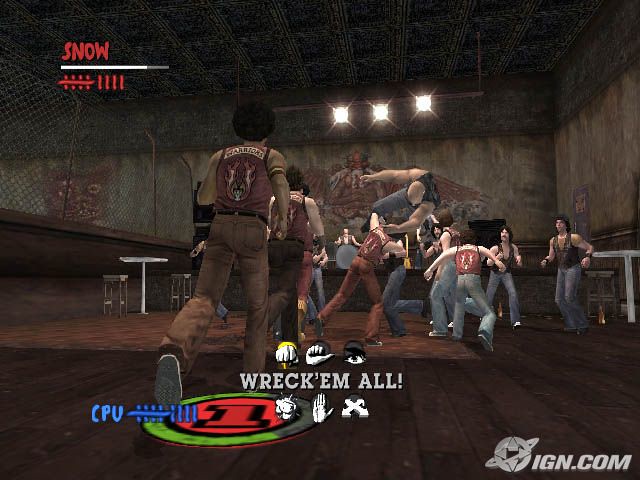The image is a detailed screenshot from a video game depicting an intense fight scene between two rival groups, likely biker gangs, indicated by their similar vests. The setting appears to be a dimly lit room that resembles a bar with a brown, camouflage-pattern interior. The room features a dark brown hardwood floor, punch tin ceiling, spotlighting, a low wall with a chain link fence, and a bar at the back accompanied by machinery and items. A large mural decorates the wall behind the bar. In the center foreground, figures with muscular builds are engaged in combat, distinguished by their attire—some wearing black muscle shirts and blue jeans, others in brown pants. The scene includes various informational overlays: at the bottom, white text reads "Wreck-Em-All!" surrounded by images of fists, hands, and swords; the bottom right corner displays an IGN.com watermark with a planet-like logo. On the right side, a green oval with a red number "1" and the word "CPU" accompanied by blue lines is present. The top of the image features three windows and the label "Snow" with a white line and ten small marks beneath it, the first four marked.